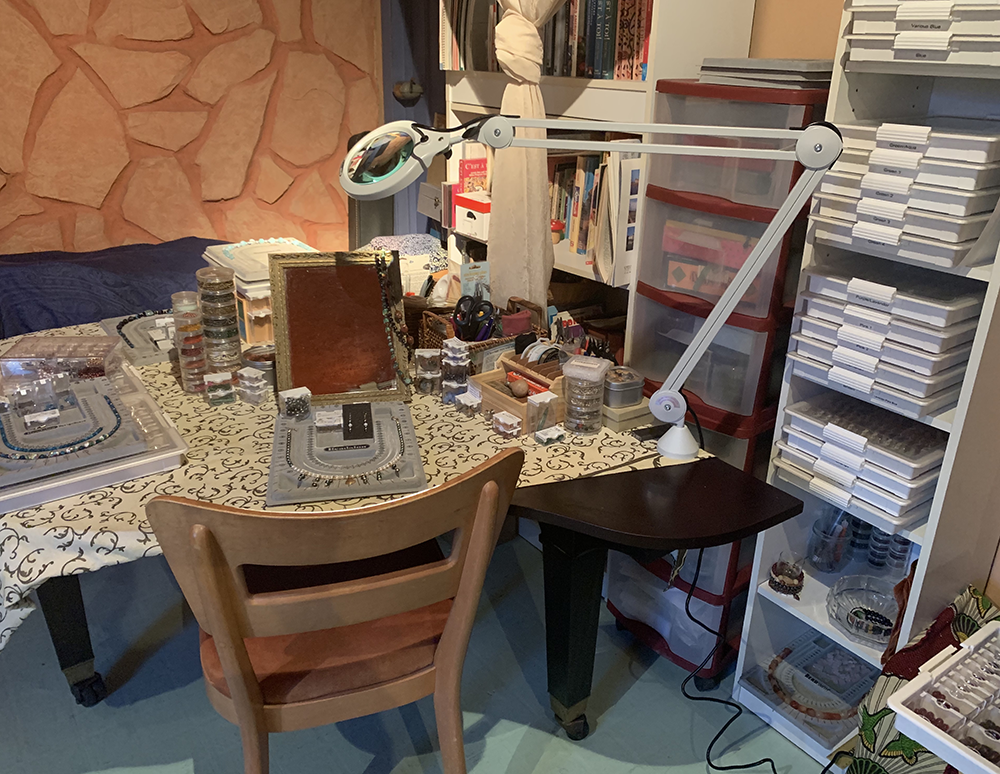The image showcases a detailed jewelry-making area, seemingly located in a basement. The backdrop features a painted, faux stone wall in a peach hue, adding a unique aesthetic to the space. On the right side, white shelves are filled with various items, including a collection of books and multiple organizers brimming with beads and assorted supplies.

The desk, situated in the middle left and center of the area, is brown and covered with a white drapery. This workspace is neatly arranged with several circular organizers containing beads in various colors such as brown, green, black, red, and yellow. Additionally, a gray template, likely used for designing necklaces, is present, showcasing different patterns and color arrangements. Another larger template is placed on the far left, indicating the creation of jewelry pieces in various sizes. A magnifying glass is also on the desk, aiding in the precision of intricate work. The overall setup reflects a well-organized and creatively inspiring jewelry-making studio.